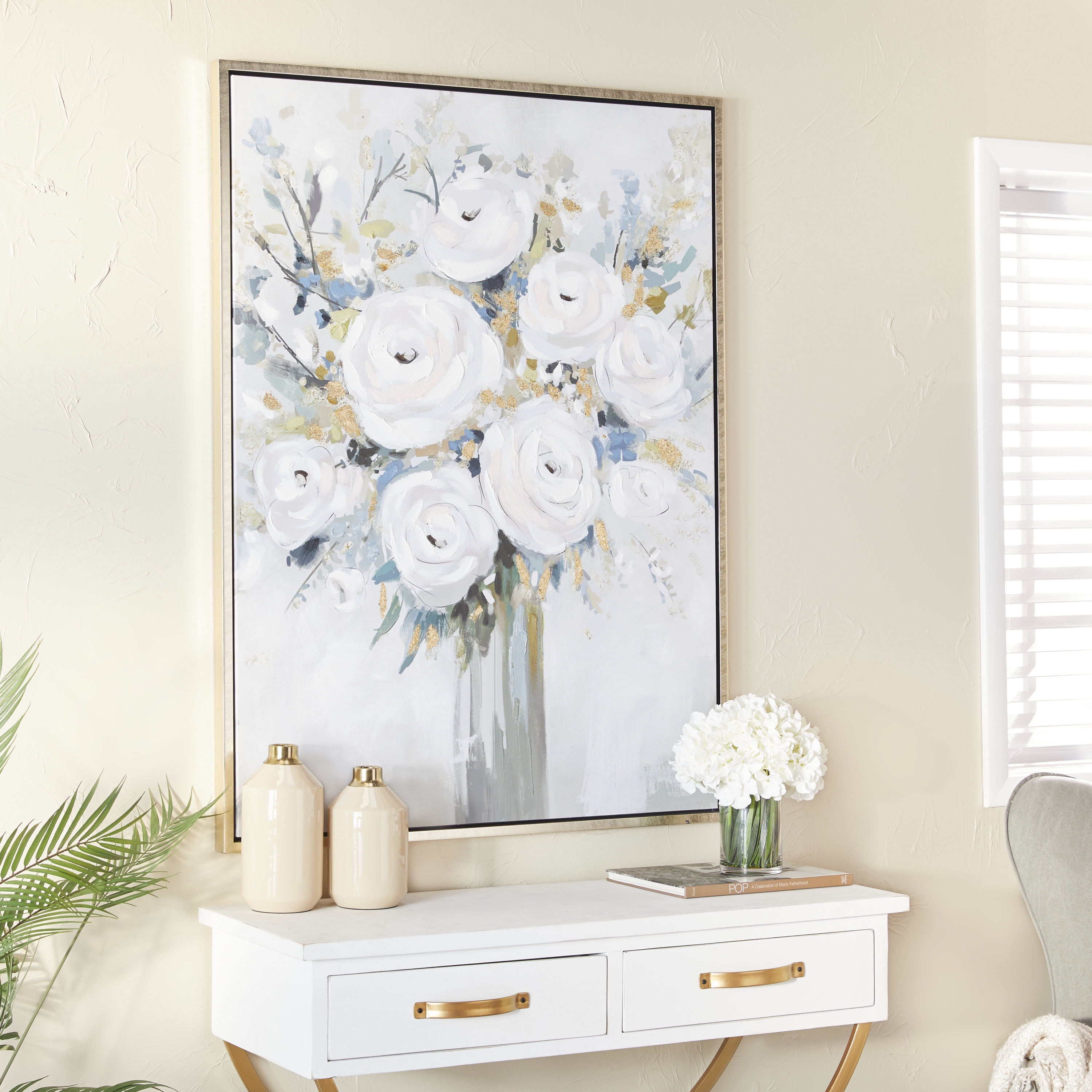This detailed photograph captures the serene ambience of a beige-walled bedroom interior. Dominating the center of the image is a large framed painting with a light wood trim, showcasing a delicate watercolor of white roses in a white vase, accented by soft blue and gold leaves against a white background. Beneath the painting is an elegant white and gold desk with two drawers; its gold handles and legs add a touch of sophistication. On the left side of the desk are two matching ivory and gold jars, with one slightly taller than the other. To the right, a small glass vase filled with white flowers sits atop a book with indistinguishable text. To the left of the image, partially cut off, are green leaves from a houseplant. On the right side, a window with partially opened blinds allows light to filter through, and just below, a gray chair is slightly visible. The careful composition and muted colors lend a calming and aesthetically pleasing atmosphere to the room.